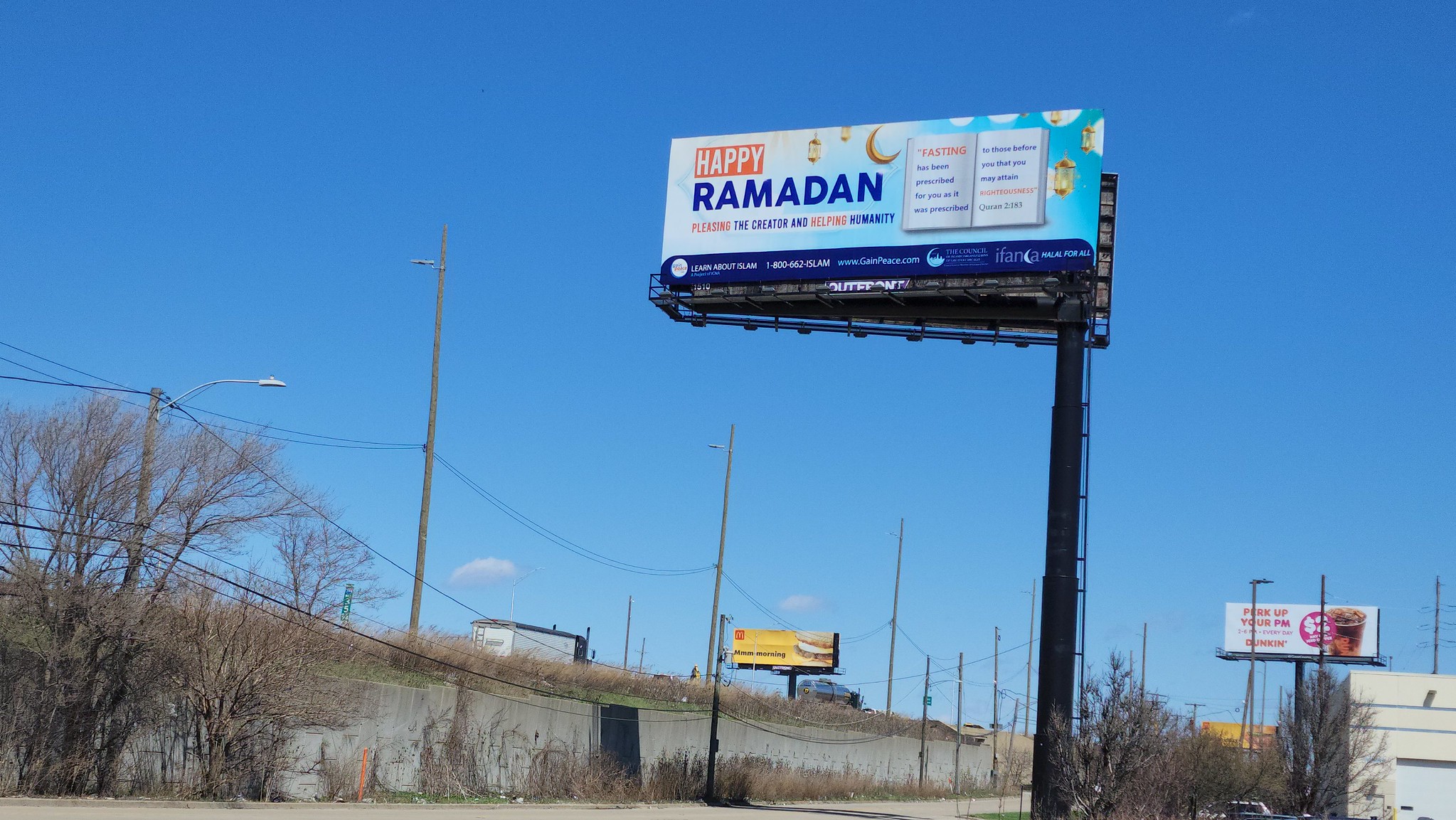The image captures a series of rectangular billboards erected on poles along a stretch of open land. The most prominent billboard in the foreground promotes "Happy Ramadan" and depicts a book titled "Moon in the Sky" set against a serene blue and white background. This rectangular advertisement is mounted on a black pole, complete with a ladder attached to its side for access. Another billboard is faintly visible behind it, though its details are obscured due to the angle. In the distance, a vibrant yellow billboard advertises a burger, while to its right, a white billboard displays an advertisement for a drink. Running parallel to these billboards is a series of telegraph poles and a road. The scene is bordered by sparse trees devoid of leaves, under a clear, bright blue sky.